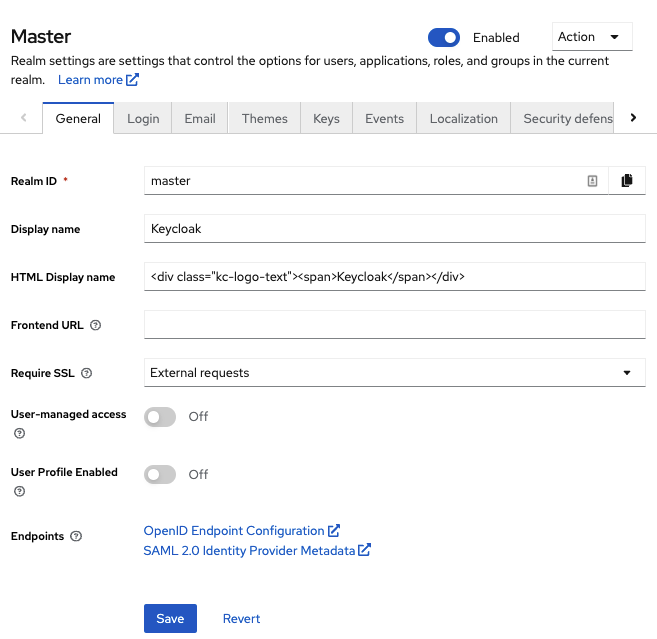This image displays the settings interface for managing various realm options. The interface includes a navigation menu with categories such as General, Login, Email, Themes, Keys, Events, Localization, and Security Defense. 

On the page, there is text explaining that realm settings control options for users, applications, roles, and groups within the current realm. The section appears to be titled "Realm ID: Master" with a display name field labeled "Master," and additional fields for the Front End URL and other configuration settings like "Keep Loook," "Require SSL," and "External Request." 

Additional settings indicate that "User Managed Access" is turned off and "User Profile Enabled" is also off. The section labeled "Endpoint" provides options for Open ID and Endpoint Configuration. There are action buttons at the bottom of the interface for saving or reverting changes made to the settings.

An option titled "Learn More" provides additional informational resources, and various toggles and buttons indicate the states or availability of certain configurable features.